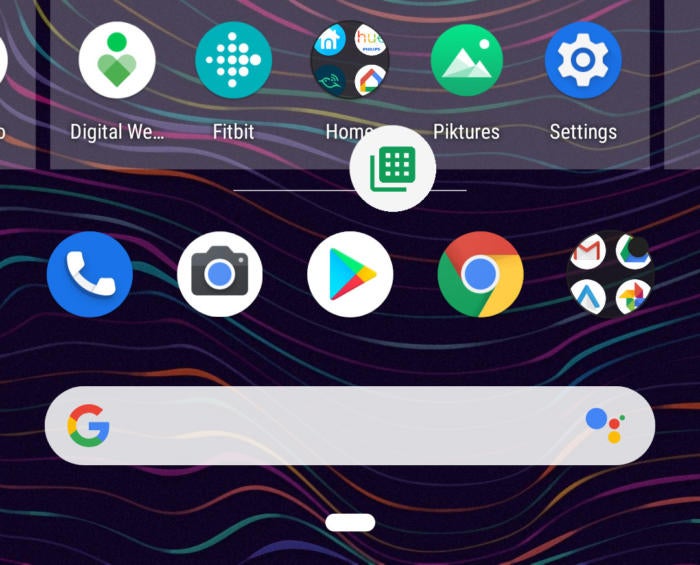The image features a vibrant and dynamic background, with swirling gradients of orange, blue, purple, and yellow creating a mesmerizing pattern. At the top left, a semi-transparent white rectangle partially reveals a circle and the word "digital," fading into an ellipsis. Adjacent to it, another semi-transparent white rectangle contains a white circle with a green circle and a green heart inside, also bearing the text "digital we...". 

Next to these elements is a blue circle filled with multiple white circles, featuring the word "Fitbit". A nearby black circle showcases a house icon, the Google symbol, and a few other icons, with partly obscured text that likely reads "home". 

Further along, a green circle with two triangles (the left taller than the right) and a circle inside presents the text "Pictures". A blue circle with a gear icon denotes "settings".

Overlaying these graphics, a white circle contains a green square composed of smaller light green squares, intersected by perpendicular lines, adding a layer of complexity. A blue circle with a phone icon, a white circle with a camera icon, and another white circle with a colorful triangle of blue, green, red, and yellow segments are scattered amongst the elements. 

The Chrome logo appears prominently, along with a collection of symbols that are difficult to distinguish. 

At the center, there’s a white rectangle with bulges on the sides, featuring the Google "G" logo flanked by a large blue dot, a smaller red dot, a small yellow dot, and an even smaller green dot. Below this, another similarly bulging white rectangle is noticeable, further contributing to the collage of digital elements.